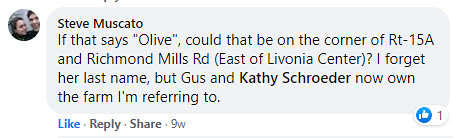This is a detailed screenshot of a Facebook comment by Steve Muscato. On the left side of the comment, there is a small, circular profile picture featuring a man and a woman. Steve's comment reads, "If that says 'Olive,' could that be on the corner of Route 15A and Richmond Mills Road, east of Livonia Center? I forget her last name, but Gus and Kathy Schroeder now own the farm I'm referring to." The comment has been liked by one person, as indicated by a small white thumbs-up icon inside a blue circle with the number "1" next to it. Below the comment, there are interactive buttons labeled "Like," "Reply," and "Share." The comment was posted nine weeks prior to the time the screenshot was taken.